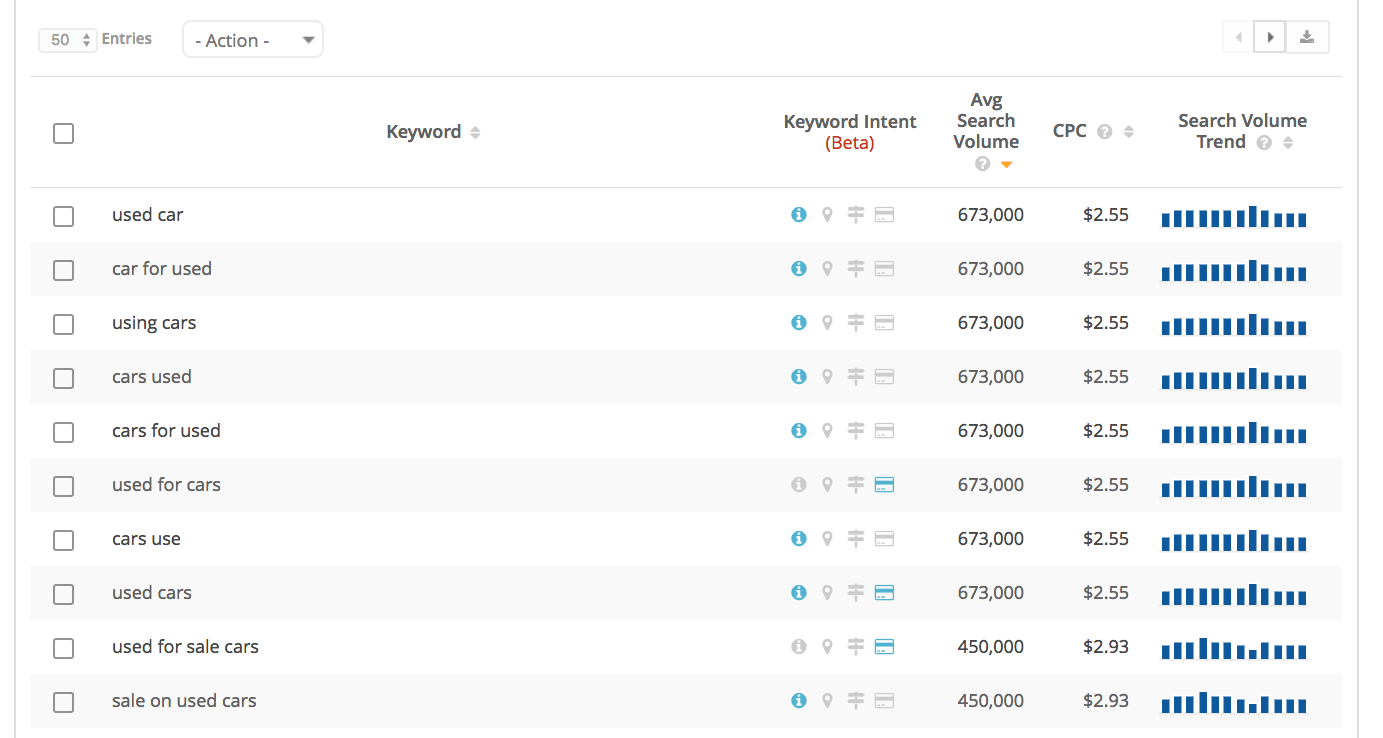**Caption:**
In the left corner of the image, there is a small box with the number "50" inside, followed by the word "entries." Next to it, inside a small box, is the word "action" with a downward-pointing arrow. Adjacent to this, there is a small square. To the right of these elements, the word "keyword" is displayed.

Below this square is a list of various categories, each accompanied by its own square checkbox. The categories include: "used car," "car for used," "using cars," "cars used," "cars for used," "used for cars," "cars use," "used cars," "used for sale cars," and "sale unused cars."

At the top, aligned with the keyword section, the words "keyword intent" are displayed with "beta" in red parentheses below it. Adjacent to this, the term "average search volume" is shown, indicating volume numbers starting at 673,000 and decreasing to 450,000 for the last two categories. 

Above this section, another category labeled "CPC" lists the cost per click for the keywords, starting at $2.55, except for the last two entries which are $2.93. Finally, on the rightmost side, under the heading "search volume trend," there is an area with about 12 short, dark blue lines placed closely together, representing the trend visually.